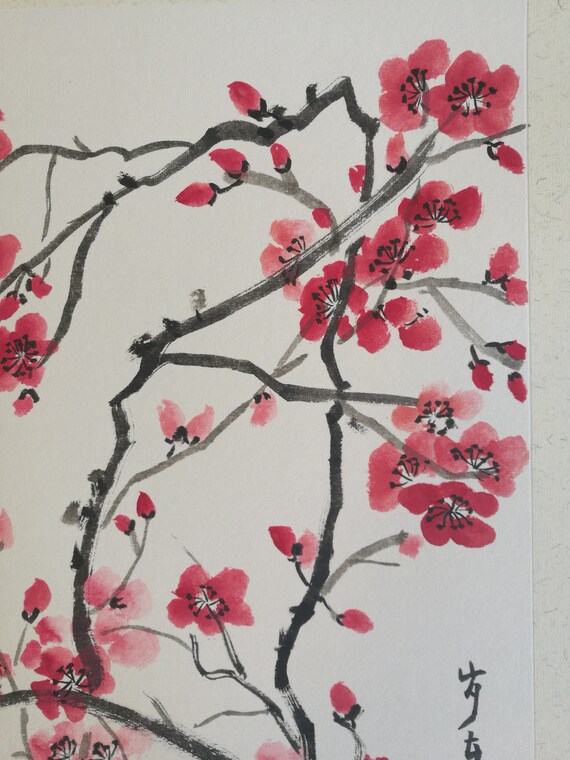The image showcases a delicate Japanese-style watercolor painting of cherry blossoms. The flowers feature pink petals, ranging from three to five per bloom, and some smaller buds that haven't yet opened. These blossoms are depicted on branches and stems rendered in shades of black and gray, achieved with single, expressive brushstrokes that lend a varied texture. The composition rests against a white-gray background, maintaining simplicity and focus on the floral elements. Japanese characters in black are inscribed on the bottom right of the painting, reinforcing the traditional aesthetic. The overall scene is minimalistic, with colors limited to the pink of the blossom petals and the monochromatic tones of the branches and background.